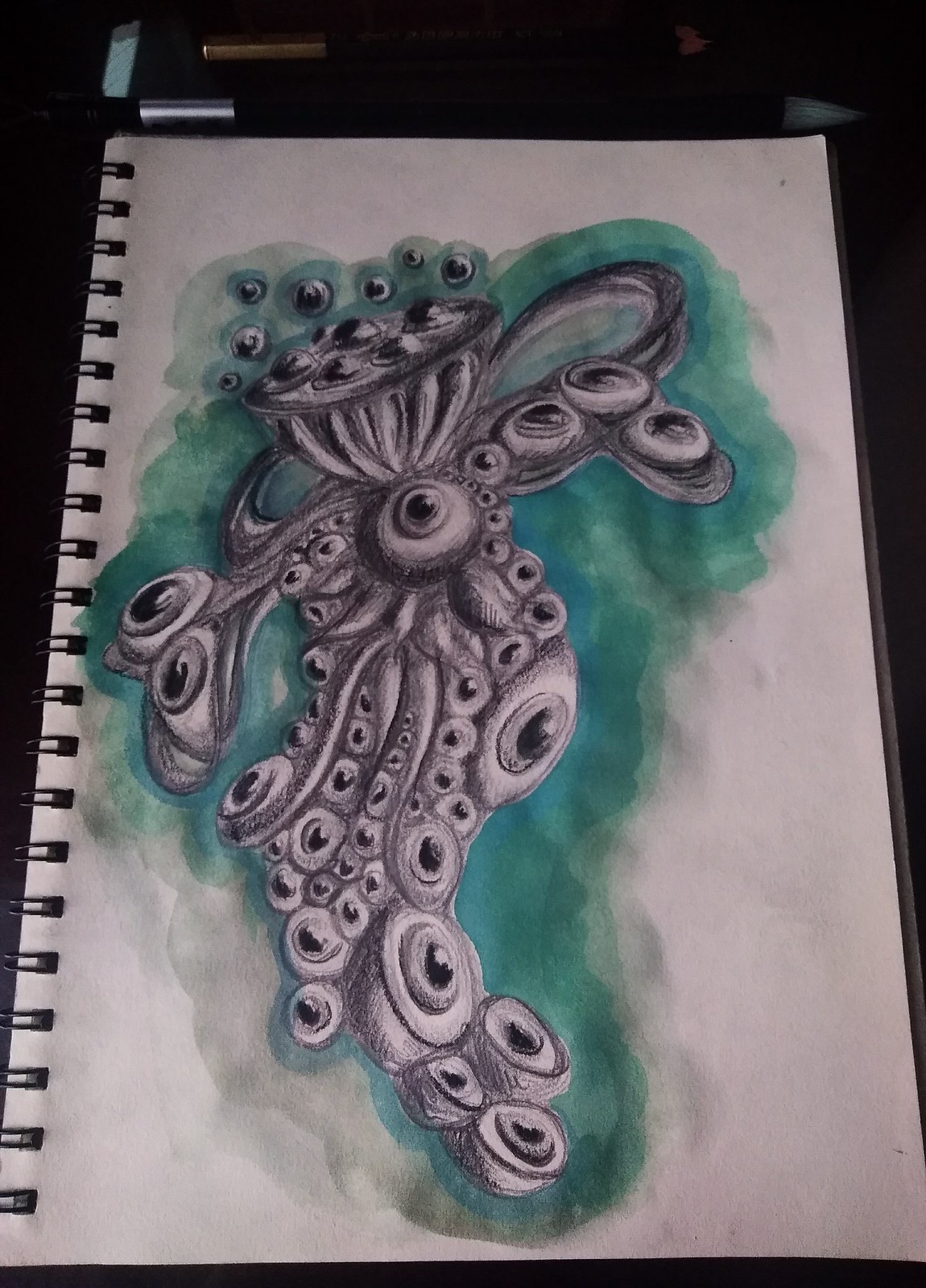This intriguing, somewhat eerie illustration appears to be created with markers or possibly paint on a piece of notebook paper that is still within the notebook. The central figure is enveloped in a swirling, mist-like formation of blue and green hues, resembling a cloud. What stands out the most are the numerous eyes embedded in this central form, each varying in size and orientation, giving the piece a hauntingly surreal quality. The composition is detailed, with the eyes seeming to peer in every direction, adding to the unsettling atmosphere. Additionally, there's a pen visible on the desk in the frame, suggesting the image was captured in an authentic, casual setting.